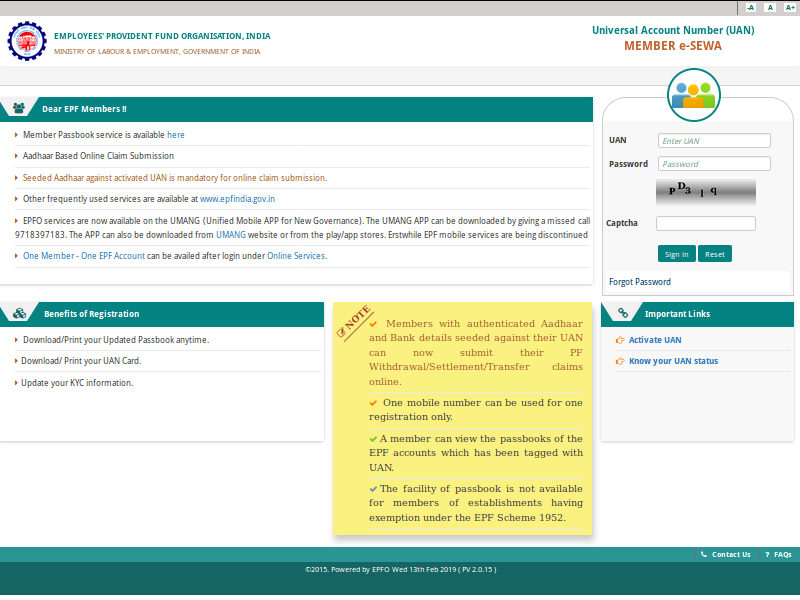At the top of the image, there is a gray border with a thin black line serving as an additional border. Just below the gray area, the background turns white. On the left side, in bright blue, capitalized bold letters, it reads "Employees Provident Fund Organization India." Below this, in brown, capitalized non-bold font, it states "Ministry of Labor and Employment, Government of India."

On the right side, in the same bright blue font, it says "Universal Account Number (UAN)." Beneath this, in a larger, bold brown font, it reads "Member E-S-E-W-A."

Underneath, there's another light gray section. Towards the right, it features an overlay of a circular white icon with a dark blue border, containing three different silhouettes. The central silhouette is orange, the one on the left is blue, and the one on the right is green.

The image then transitions into a rounded rectangular area. The top part has a white background, shifting into a light gray background. In bold, capitalized black letters on the left, it reads "UAN," beside an editable field with the placeholder text "enter LAN or LIAN" in small, italicized, bluish font.

Below this, towards the left, it says "Password" in bold black letters, with an adjacent field for entering the password. There is a captcha section below this, with a corresponding field to enter the captcha code. 

At the bottom of this area are two rectangular buttons: the left button says "Sign In" and the right button says "Reset." Both buttons have a dark teal green background with white font. Towards the bottom left of the image, in bold blue font, it says "Forgot Password."